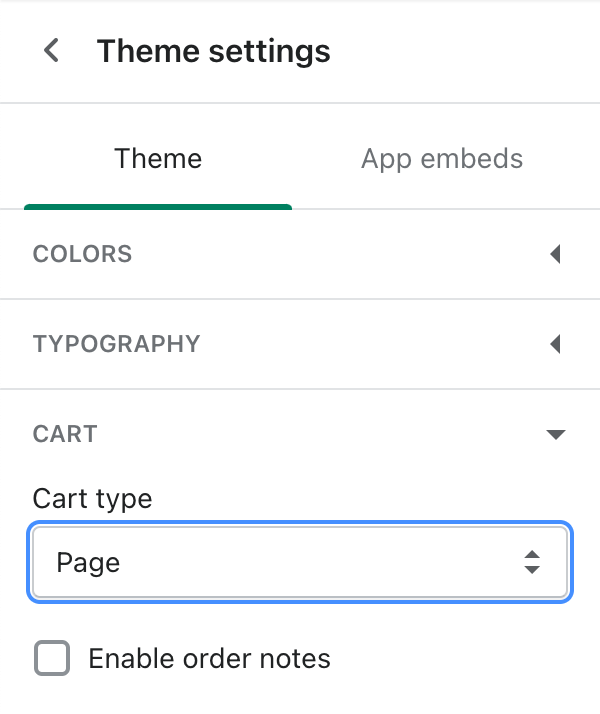The screenshot features an Android phone displaying the theme settings page. In the upper left corner, there is a gray "less than" symbol (<) indicating a back option. To its right, "Theme Settings" is displayed. The top of the screen is bordered by a light gray horizontal line, with a darker horizontal line at the bottom of the header.

The primary section below is labeled "Theme" in bold black text, underlined with a green horizontal line. Next to "Theme," "App Embeds" is shown in gray text, separated by another green horizontal line.

The following section, titled "COLORS" in all capital letters, features gray font. To the right of the heading is a small left-pointing gray triangle, separated by another horizontal gray line.

Continuing down, the next heading reads "TYPOGRAPHY" in all capital gray letters, accompanied by a small gray triangle pointing to the left on the right-hand side.

Further down, the label "CART" appears in all capital gray letters with a downward-pointing gray triangle on the right. It is followed by the label "Cart Type" in black text. Below this, a blue-highlighted rectangle contains the word "Page," flanked by up and down triangles indicating a drop-down menu. An option to "Enable Order Notes" is available at the bottom of the screenshot.